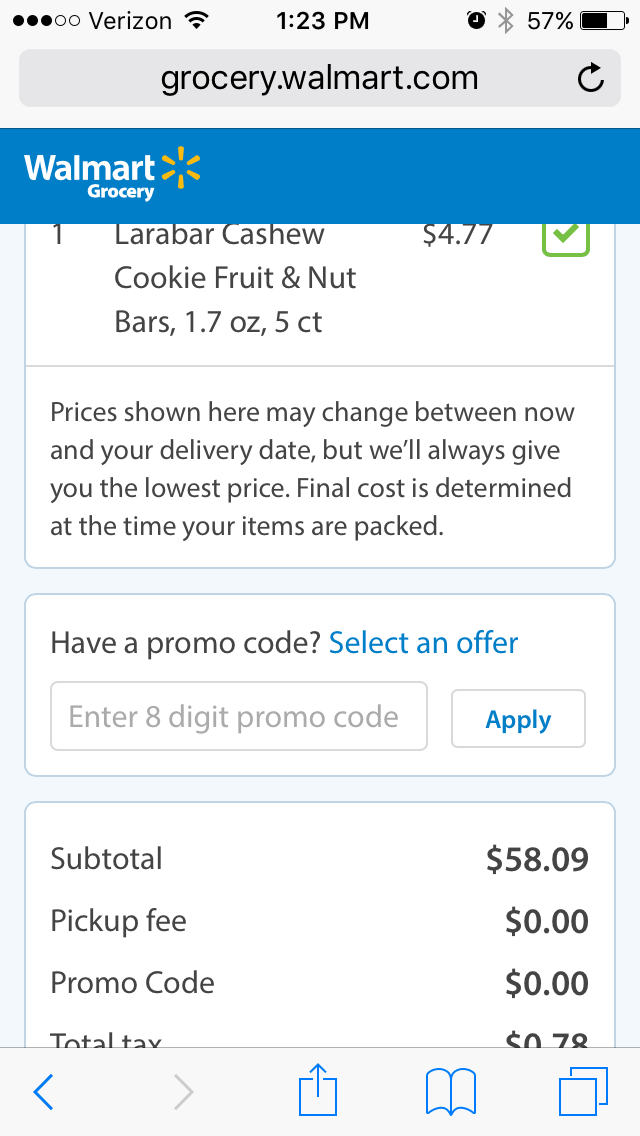The image displays the Walmart grocery website on an iPhone. The web address is grocery.walmart.com, showcasing the mobile interface of the online grocery service. The status bar at the top indicates that the device is connected to Verizon with three out of five signal bars, and Wi-Fi is at full strength. The time displayed is 1:23 p.m. Additional icons include an alarm symbol, a Bluetooth symbol, and a battery life indicator showing 57%.

The shopping cart section highlights one item: a Larabar Cashew, priced at $4.77. The item is specified as "Cookie, Fruit, and Nut Bars," weighing 1.7 ounces with a count of five. A green check mark confirms the item is in stock.

A message informs users that prices may change before the delivery date, but Walmart will provide the lowest price, with final costs determined upon packaging. Options to enter a promo code are available, with a noted subtotal of $58.09, a pickup fee of $0, a promo code value of $0, and a total tax of $0.78.

Below the cart details, buttons for sharing, bookmarking, and managing multiple browser tabs are visible.